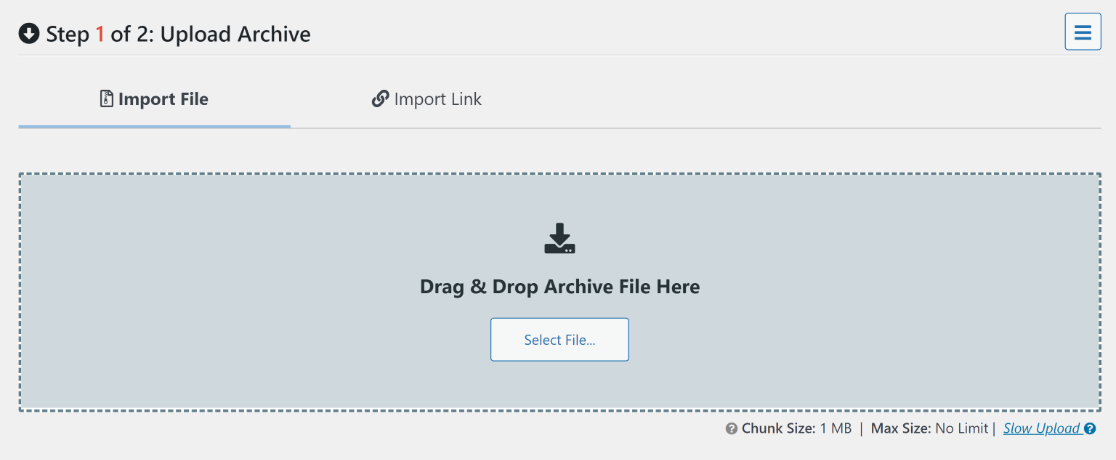The image depicts a computer screen displaying a web page with a predominantly light gray background. Centrally positioned is a darker gray box. At the top of the screen, the text "Step 1 of 2: Upload Archive" is clearly visible, indicating the beginning of a multi-step process. Below this header, there are two options: "Import File" and "Import Link." The highlighted or selected option is "Import File."

Inside the darker gray box, a prompt reads "Drag-and-drop archive file here," suggesting an area for users to upload files. Additionally, there is a smaller white box with the instructions "Select File," which likely functions as a clickable button for file selection.

Located at the bottom right corner of the interface are details about upload limitations: "Chunk size 1 MB, Max size no limit," implying the maximum size of the upload is unrestricted, though individual file chunks are processed in 1 MB increments. To the far right of these details, the term "Slow Upload" appears alongside a small question mark icon, which users can click for more information about what "slow upload" entails.